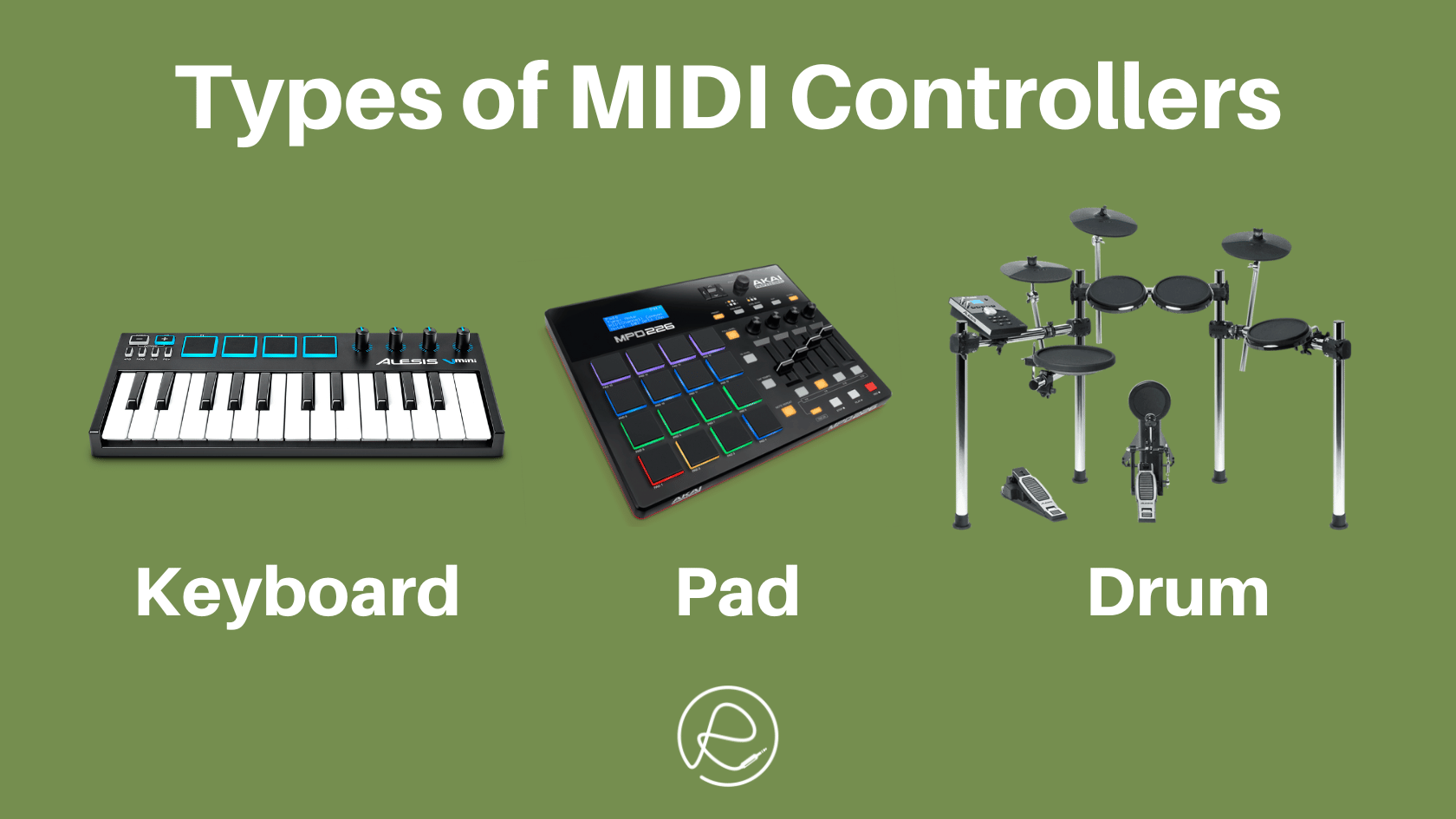The image presents a detailed informational chart against an olive green background, titled "Types of M.I.D.I. Controllers" in light beige text at the top. The bottom section features three distinct images and labels. On the far left, a modern keyboard is depicted in black and white, with the label "Keyboard" written beneath it in matching light beige. The middle image shows a rectangular electronic pad, predominantly black with colorful buttons in red, green, and blue, labeled "Pad". To the right, an electronic drum set is displayed in predominantly black and gray tones, labeled "Drum". Additionally, at the lower third of the page, there is a circular symbol with a hand-drawn "R" in the center.